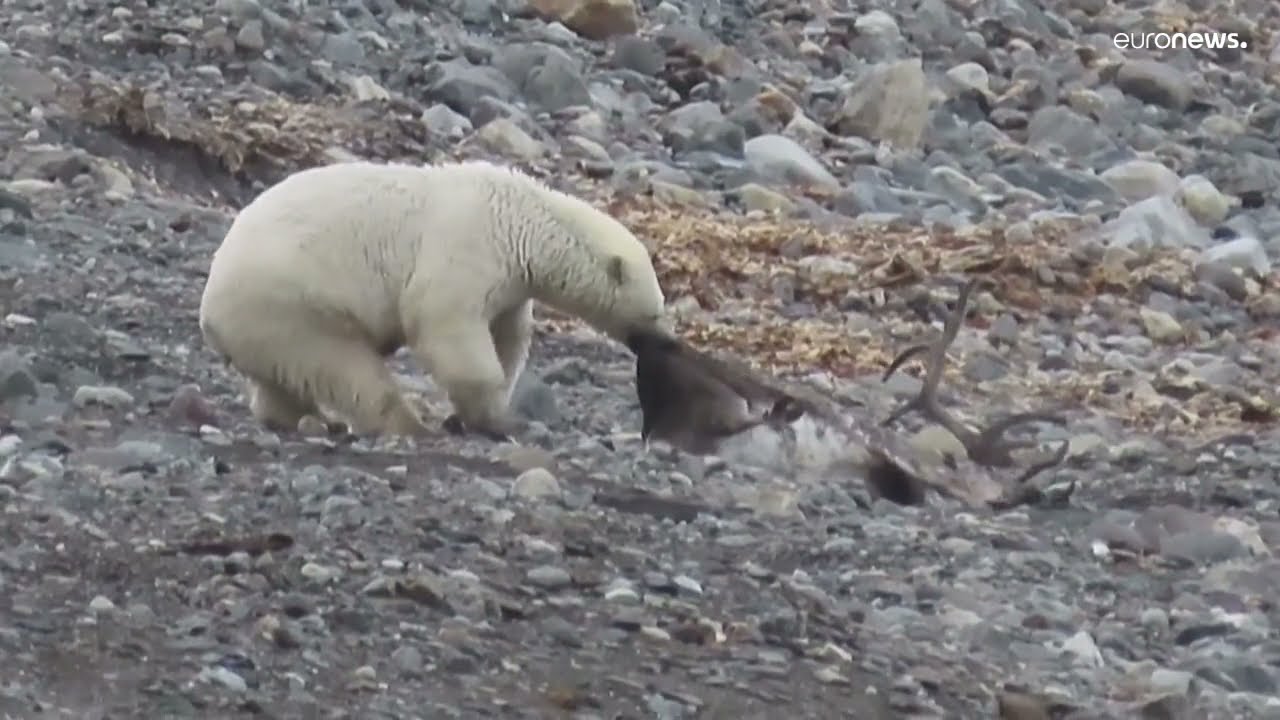In a rugged, rocky landscape captured in the wilderness, a polar bear with matted and slightly darker fur, especially around its hind legs and forepaws, is seen tugging at a carcass. The scene is dominated by rocks of various sizes and shades, ranging from gray to brown, with exposed patches of brown dirt creating a stark backdrop. The polar bear, positioned on the left side, uses its mouth to drag a dead elk, identifiable by its prominent brown antlers, which is lying on the ground on the right. The elk's fur exhibits a mix of brown on its sides and white on its chest. The top right corner of the image bears the text "Euro News," indicating the source of this dramatic nature capture.